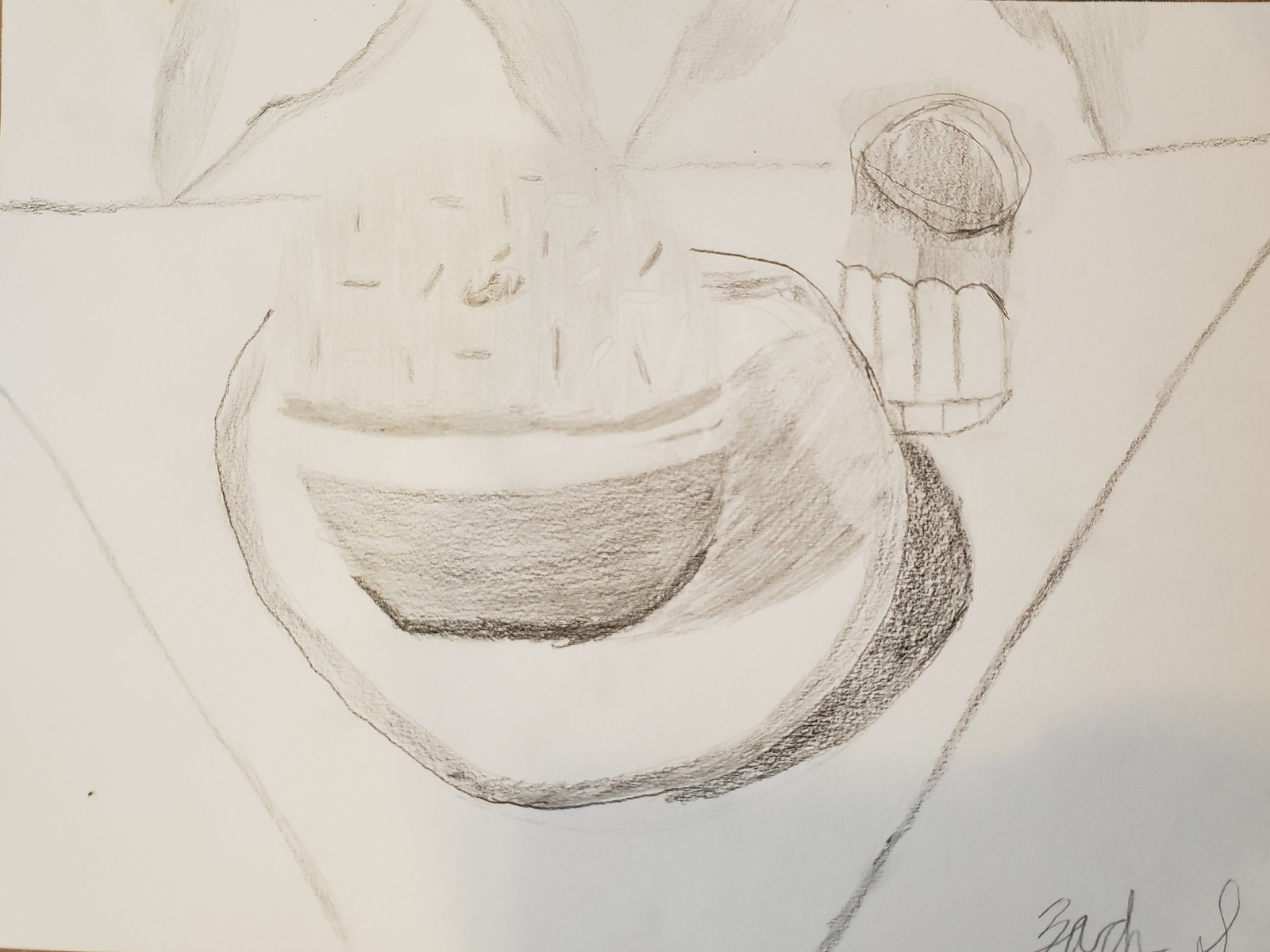This black-and-white charcoal drawing features a rabbit as its central subject, though the depiction is somewhat abstract, making it challenging to identify at first glance. The artist's signature is located in the lower right corner and appears to start with the letters "B," "A," "D," possibly forming the name "Badel" or a similar variant. The composition includes two lines originating from the bottom and extending upward to form a triangular shape, which seems to represent the rabbit's ears. In the middle of the drawing, there is a circular object, possibly a can, and an outline resembling the head of the rabbit, imbued with a mouth. The abstract nature of the artwork lends a unique, interpretative quality, inviting viewers to explore the nuances and textures created by the charcoal medium.